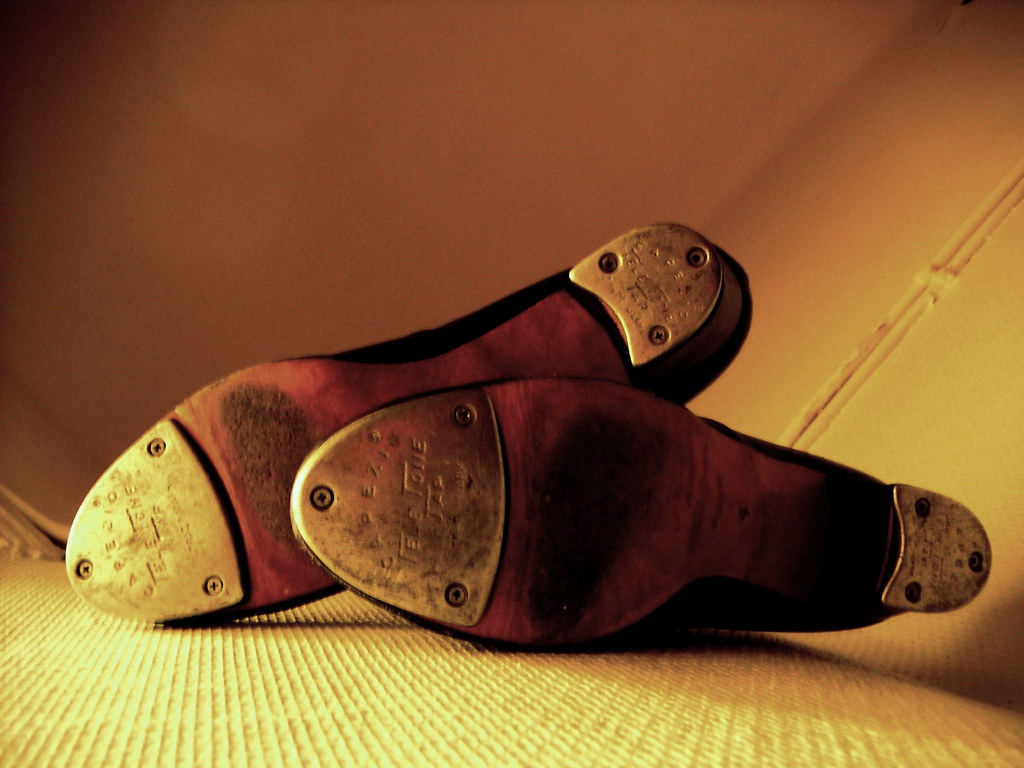This horizontal rectangular photograph showcases the aged and dirty bottoms of a pair of tap shoes, clearly identifiable by the metal plates secured with three Phillips head screws on both the toe and heel. The shoes, resting on their side on a textured cloth base that resembles a car seat or some undefinable leather strip, exhibit traditional medium brown leather soles heavily worn with dirt. One shoe points west, while the other leans upward, both featuring metal plates—one likely gold or silver in color. Though partially obscured by shadows, the tops of the shoes appear to be black. The front tap metal plate bears a worn logo that reads "Capezio Teletone Tap."